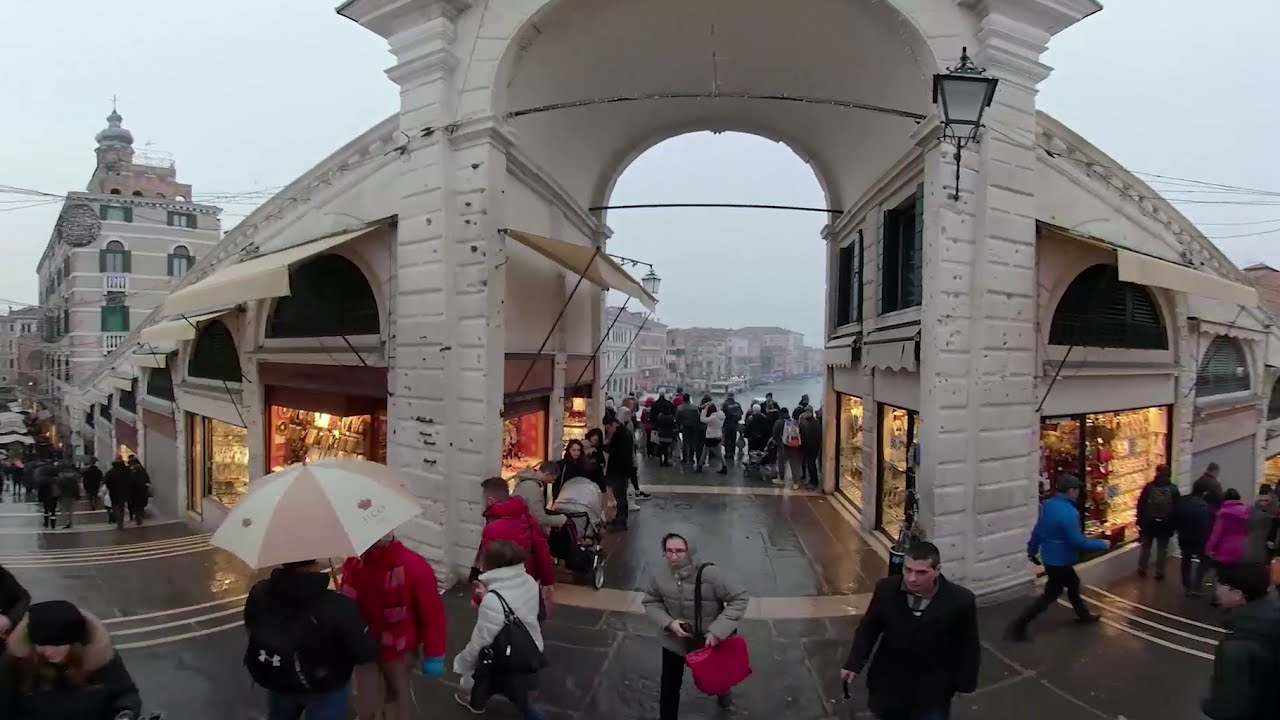The image captures a bustling outdoor mall with a grand white granite or white brick archway at its center, flanked by well-lit shops with awnings. The scene is lively, with over 100 people walking in various directions, including a family with a baby carriage and an umbrella-covered couple in red down jackets, suggesting it is chilly and raining. People are dressed in coats, and many are holding umbrellas. Beyond the arch, a group of people stands, some gazing out towards what appears to be a lake or canal in the background. The photo is taken in a city setting, possibly during late afternoon or early evening, as suggested by the well-lit stores and the gathering crowd.